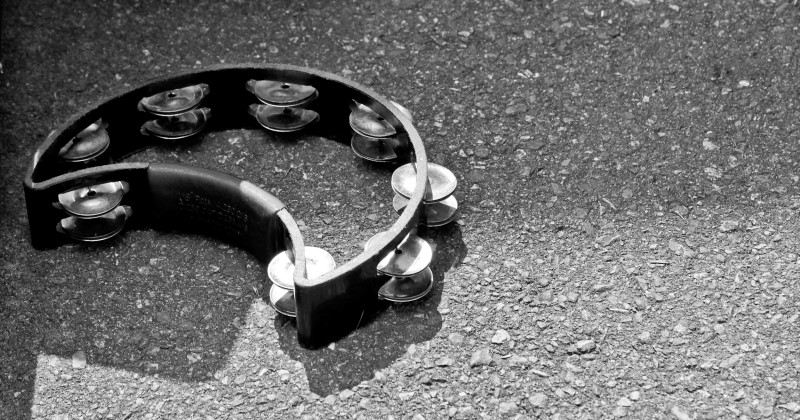In this black and white image, a crescent-shaped tambourine with a handle designed for handholding lies on a grainy surface that appears to be stone-paved asphalt. The pavement features a slightly rough texture with small, inset pebbles of varying shades that form a generally smooth surface. The tambourine itself is dark in color, contrasted by lighter metallic cymbals arranged in pairs along its half-circle body—six pairs along the curved edge and two near the handle, which together resemble a crescent moon. The light source casts a shadow on the top left, with the asphalt appearing lighter in the bottom right. Some of the metallic cymbals show subtle reflection marks, adding a touch of brightness to the otherwise monochromatic scene.